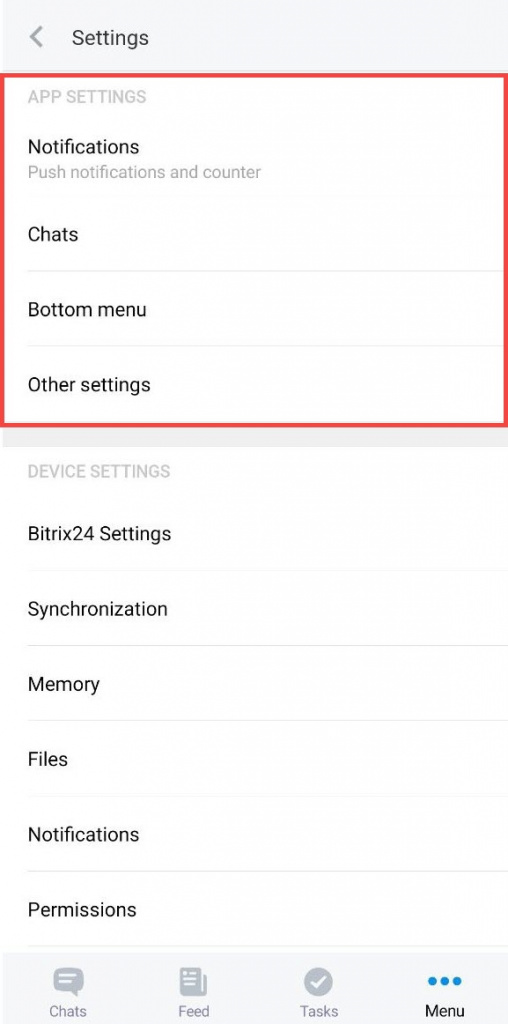The screenshot displays a settings menu from a mobile application. At the top, there's a gray border, with a left-facing triangle icon labeled "Settings." Below, within a red-outlined white box, the section is titled "App Settings," offering four options. The first option, "Notifications," includes "Push Notifications and Counter." Following that, the other choices listed are "Chats," "Bottom Menu," and "Other Settings."

A light gray line separates this from the next section titled "Device Settings," presented in light gray text. Underneath, the "Bittrex 24 Settings" are detailed with sub-categories: "Synchronization," "Memory," "Files," "Notifications," and "Permissions," each divided by a similar light gray line.

At the bottom is another gray border. On the left, there's a conversation pop-up icon labeled "Chats," followed by a "Feed" option. Next, a circle with a checkmark labeled "Tasks" sits to the right of "Feed." The last item on the far right features three horizontal blue dots labeled "Menu" in black. It appears that the "Menu" option has been selected, indicated by its text being highlighted in black.